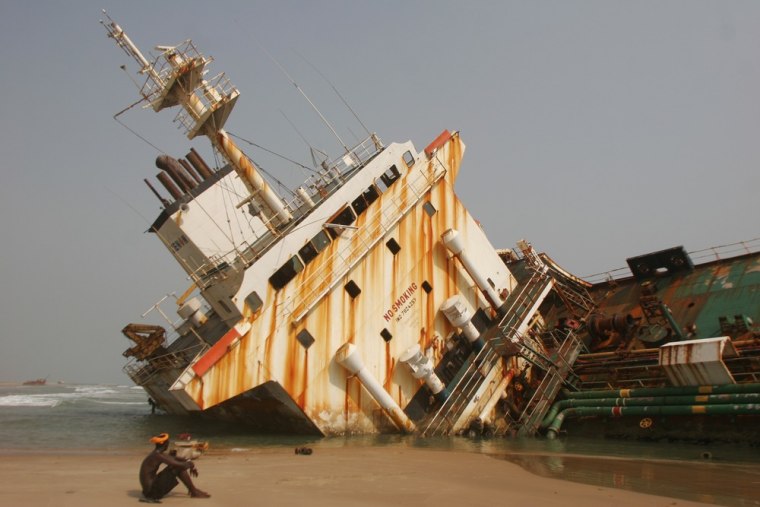The image captures a dramatic scene of a boat appearing to capsize into a muddy bank, with part of it already submerged in brown, murky water. The boat, heavily rusted with horizontal streaks of rust running down its green and white hull, is tipping over in what seems to be a shallow area, possibly quicksand. The setting is outdoors during the day, characterized by an overall bright yet grayish light, with a clear gray sky and a somewhat grayish ocean. In the bottom left corner, a man with dark brown skin sits intently watching the boat as it sinks. The scene unfolds at what resembles a beach, lending a stark, almost surreal contrast between the decaying boat and the serene beach setting.